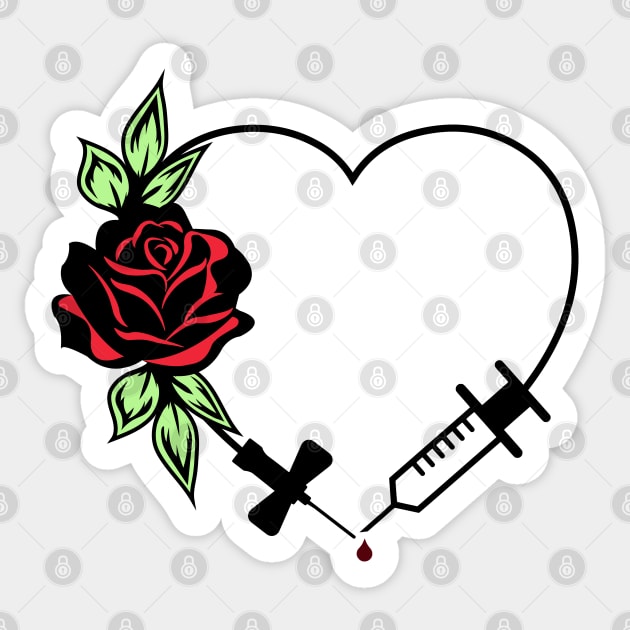The image is a color photograph featuring a detailed tattoo template shaped like a heart, occupying most of the square frame, which measures approximately four inches by four inches. The heart is outlined in black and set against a light gray background with subtle gray diamond patterns, each featuring a small gray circle with a light gray outline and a padlock inside.

At the heart's left side, a red rose in bloom is depicted, with three green leaves pointing up and three pointing down. Adjacent to the rose, forming part of the heart's outline, is the black adjustment handle of a butterfly IV needle. As the outline continues, it transforms back into a simple black line before rounding to the right, where it becomes a syringe. The syringe, detailed with an outline of the tube and a plunger, points downward and terminates with a drop of blood. This drop appears white against the gray background, with a hint of red around it.

The entire image is bordered in white, contributing to the crisp and clean photographic realism style of the artwork.